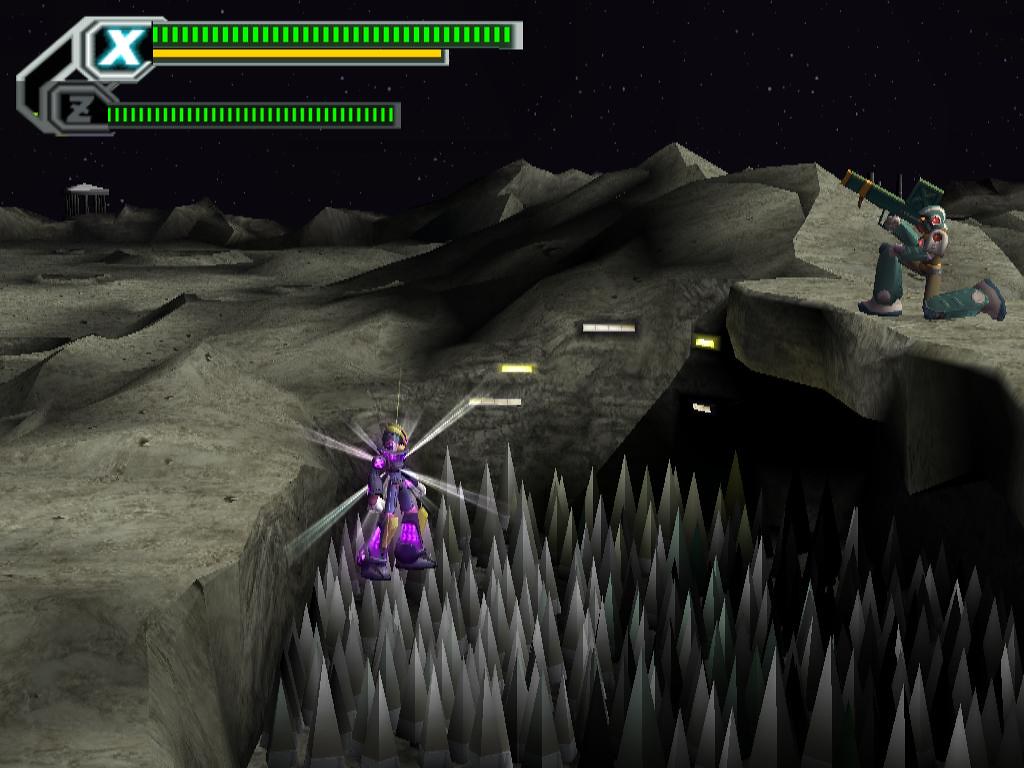This is a screen capture from a video game set on an alien planet or outer space environment. The scene displays a barren, rocky, gray terrain covered with sharp, triangular spikes in the lower right corner. The background consists of a dark black sky dotted with white stars. Two armored characters dominate the scene. One character, in a bright purple space suit with lights emanating from them, is hovering or attempting to navigate over the dangerous spike pit. The other character, clad in green and purple armor with distinct green pants and brown protective gear around the upper leg, is kneeling on a rocky ledge. This second character is aiming a large gun or weapon towards an unseen target. Additionally, green indicator bars labeled 'X' and 'Z' are visible in the upper left corner, presumably showing the characters' health status or another in-game metric. The entire setting is filled with jagged cliffs and a rugged surface, emphasizing the hostile and treacherous nature of the environment.